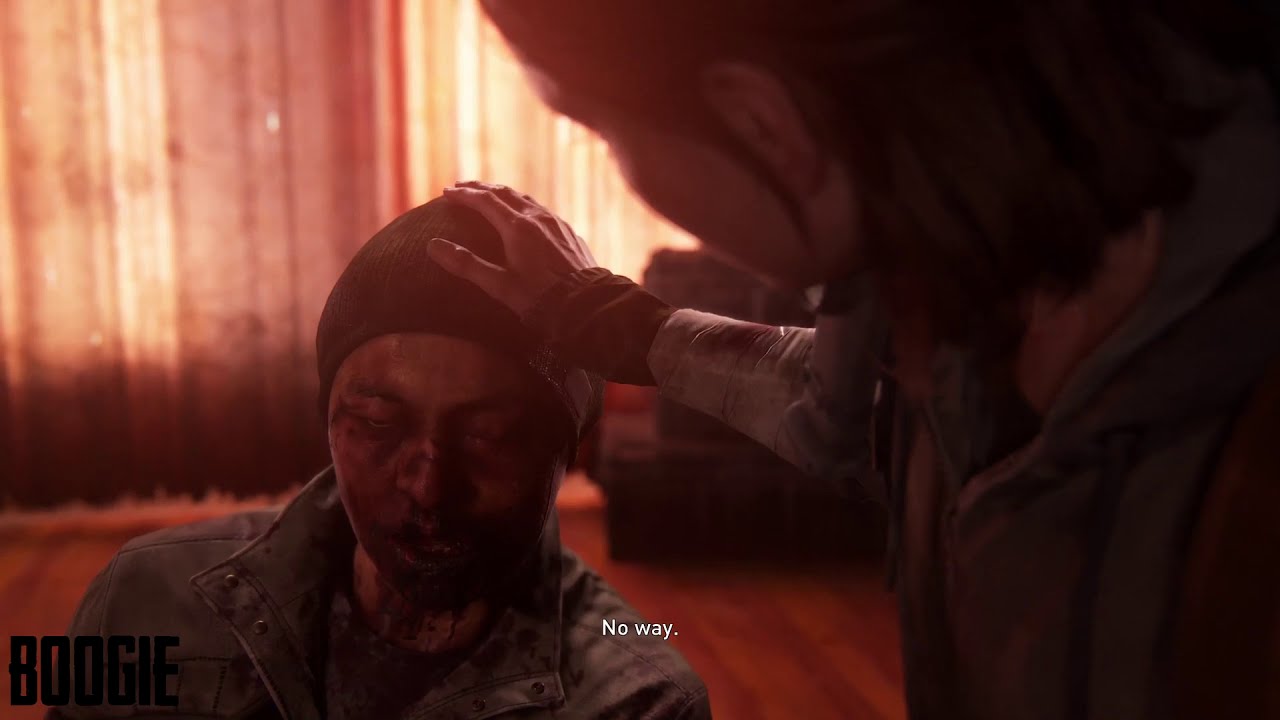The image appears to be a dramatic scene from a movie, TV series, or possibly a video game given its detailed rendering and lighting. It takes place in a dimly lit room that resembles a hotel or a residential space, characterized by dark wooden floors and large, red curtains covering the windows, casting a moody, reddish glow. 

In the foreground, a young Asian man with a swollen, bloody face and visible bruises, especially around his eyes and cheeks, sits or kneels on the floor. He wears a grey jacket stained with blood and has a beanie on his head. Blood drips from his nose and down his neck, underscoring the severity of his injuries. 

Next to him, a woman with black hair, whose face is turned away from the camera, leans over him with her hand gently placed on his head in a comforting gesture. The light from the background silhouettes her figure, making her the prominent feature on the right side of the image. 

Small, white text at the center bottom reads "No Way." In the lower left corner, the logo "Boogie" is displayed in black letters, hinting at the source or title related to this scene.